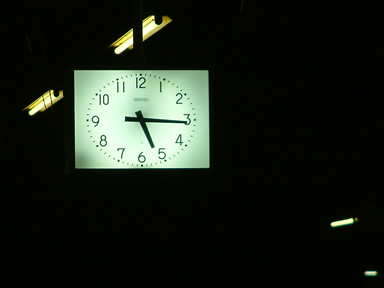This indoor photograph features a central, illuminated square displaying a clock face that reads 5:15. The square stands out starkly against a completely black background, with only a single fluorescent hanging light visible above and slightly behind the clock. The fluorescent light is turned on, casting a dim, focused glow, yet not sufficient to illuminate the surrounding area, which remains in deep darkness. The composition creates a dramatic contrast, emphasizing the clock's bright face amidst the enveloping shadows.